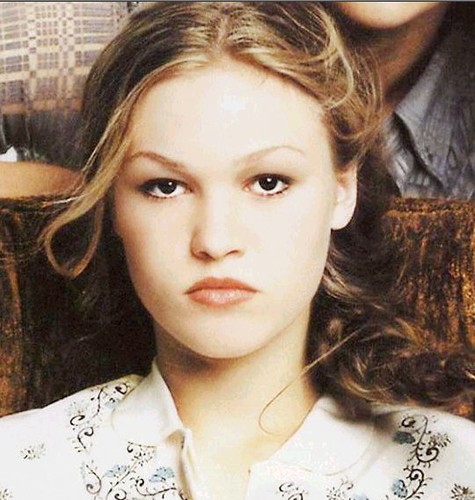The photograph is a detailed color image of a young woman, identified as actress Julia Stiles, viewed from the shoulders upwards. She sports a serious expression, with brown eyes looking directly forward. Her hair, a brownish blonde mix, is neatly pulled back, accentuating her coral lipstick. Julia wears a white blouse adorned with a turned-down collar and a variety of intricate black and blue floral and paisley patterns. The blouse’s designs consist of loopy shapes, some resembling backward S's with small floral details.

In the background, there are hints of additional individuals, partially obscured. Behind Julia, there appears to be a brown chair, possibly velvet. A neck and chin of another person can be seen, who is wearing a gray collared shirt. There is also a striped gray and white shirt visible in the background, belonging to another indistinct figure. The overall scene is composed with subtle details that add a layer of complexity and richness to the photograph.